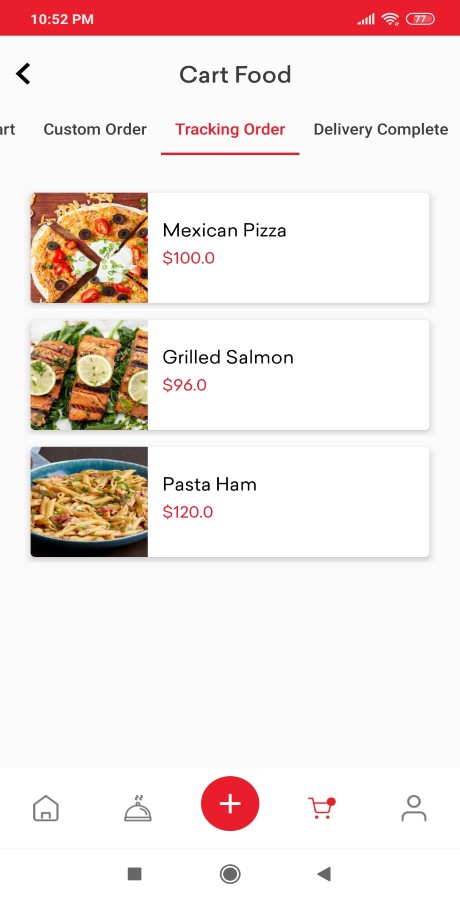The screenshot captures a cell phone interface from a food delivery app. The top of the screen features a red horizontal bar, displaying the time on the left and icons for battery, reception, and Wi-Fi on the right. Just below this bar, the background is light gray. On the left side of the screen, a bolded left arrow, resembling a sideways "V", is visible. Centered on the same line in black text, it reads "Cart Food".

Underneath, there's a navigation menu. On the left, the letters "RT" are partly visible. To the right are menu items: "Custom Order" and "Tracking Order" (highlighted and underlined in red), followed by "Delivery Complete".

Further down, the interface displays three white rectangular sections, each containing details of food items. The first rectangle features an image on the left of a Mexican pizza. To the right, it is labeled "Mexican Pizza," with its price in red below, listed as "$100.0". The second rectangle shows an image of three grilled salmon pieces with a lemon in the center. To the right, it is labeled "Grilled Salmon," priced at "$96.0" in red text below. The third rectangle features a bowl of pasta. To the right, it is labeled "Pasta Ham," with the price in red listed as "$120.0".

At the bottom, another white rectangle contains icons from left to right: a house, a service bell, a plus sign, a shopping cart, and a person, likely representing various app functionalities.